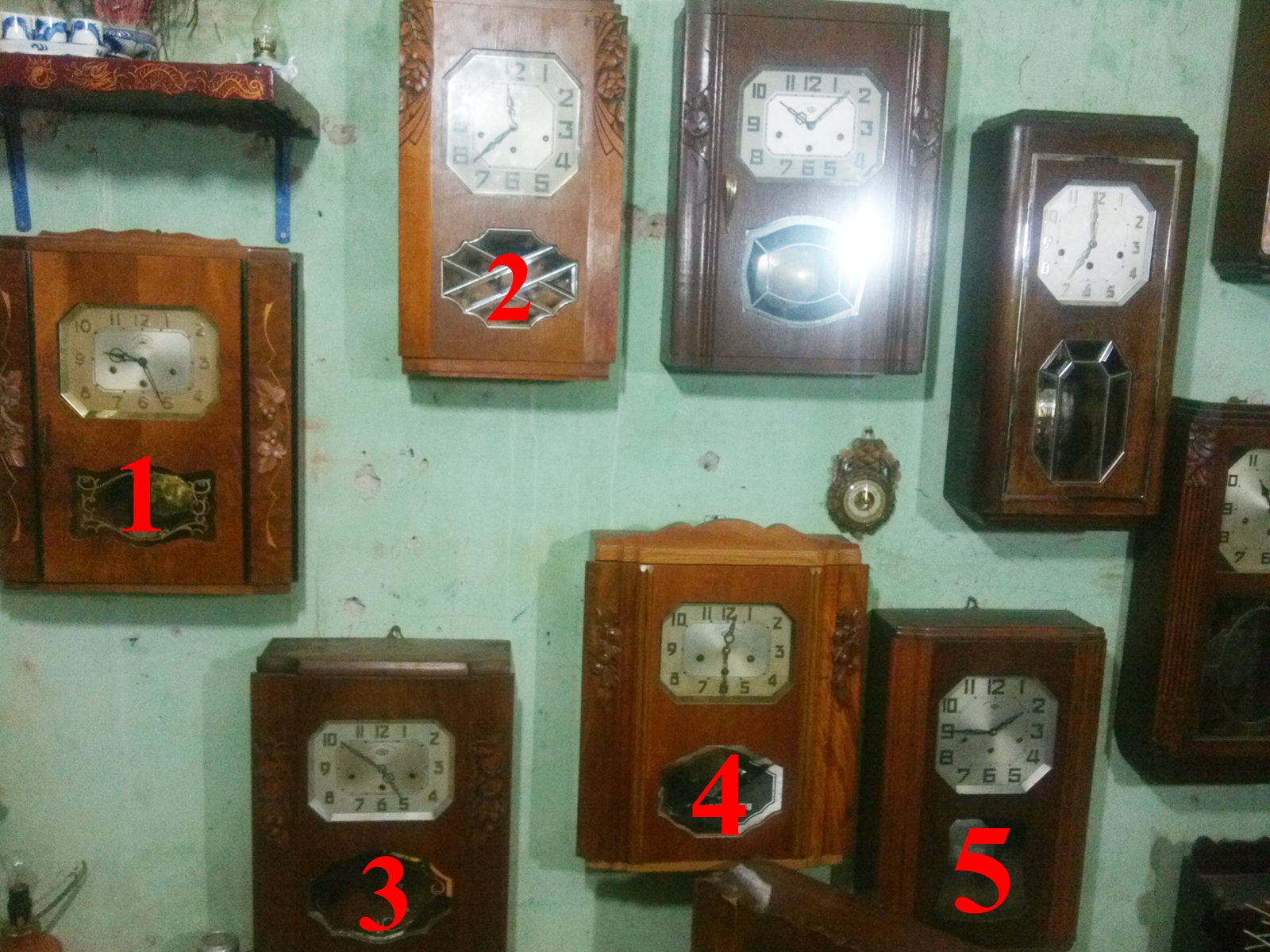The image depicts an indoor scene with several vintage clocks hanging on a tealish-green wall. These clocks, which number eight in total, are arranged in a circular pattern. They each have a box-like structure with white or gold faces and feature real numbers instead of Roman numerals. Interestingly, some of the clocks are square while others are octagonal. Only five of the clocks are digitally marked with red numbers: the far left clock is numbered 1, the one up and to the right of it is numbered 2, and at the bottom left corner, clocks numbered 3, 4, and 5 are arranged in sequence moving rightward. The remaining three clocks are unnumbered. The clocks appear to resemble plaques at the bottom and vary slightly in shape, adding a vintage charm to the display.